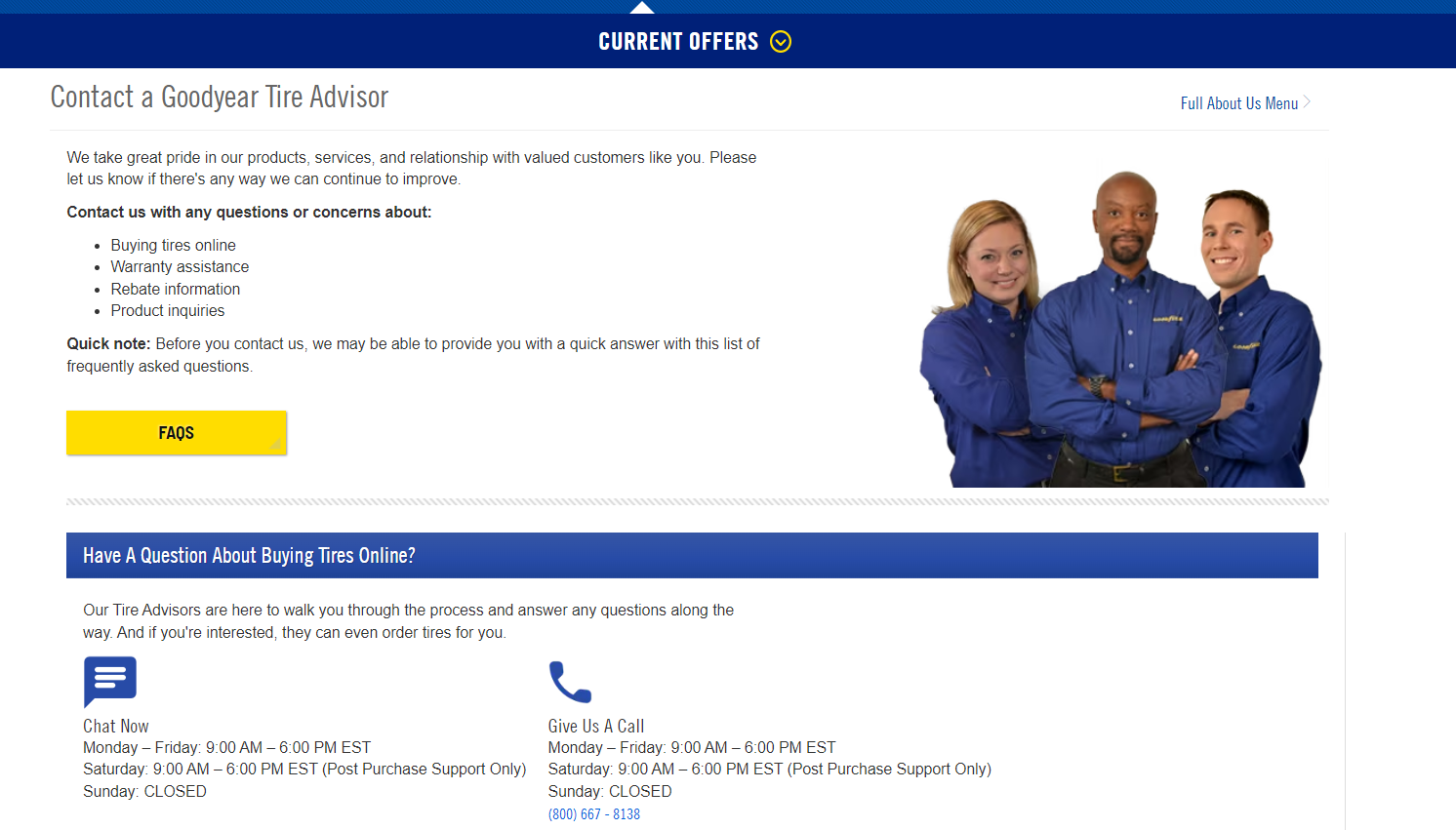A detailed and cleaned-up caption for this image could be:

---

The image is a screenshot from a company's website. At the very top, a thin blue border with a triangle pointing upwards suggests it may be clickable for additional information. Below this, a wider blue bar features the text "Current Offers" in a dark white font, accompanied by a blue circle with a yellow border and a check mark inside it.

The central section, featuring a white background, occupies about half the page and highlights the message: "Contact a Goodyear Tire Advisor. We take great pride in our products, services, and relationships with valued customers like you. Please let us know if there's any way we can continue to improve. Contact us with any questions or concerns about:" followed by bullet points for buying tires online, warranty assistance, rebate information, and product inquiries.

A yellow box labeled "FAQs" suggests checking frequently asked questions for quick answers. 

To the right, a header reads "FULL About Us Menu" in blue, prefaced by a right-pointing caret. Below this is an image of three young individuals in their 20s or 30s: a white woman with long blondish-brown hair, a Black man with a bald head, thin mustache, and goatee, and a smiling white man with short dark hair. All three are wearing blue button-down shirts emblazoned with the Goodyear emblem on the upper right chest and have their arms crossed.

Beneath the image, a small blue-lined bar introduces the section: "Have a question about buying tires online?" The text continues: "Our tire advisors are here to walk you through the process and answer any questions along the way. If you're interested, they can even order tires for you." The section also includes a chat box with "Chat Now" written on it, indicating available hours: Monday to Friday, 9 a.m. to 6 p.m. EST, and Saturday, 9 a.m. to 6 p.m. EST (post-purchase support only). It is closed on Sundays.

Adjacent to this, a phone icon accompanies the invitation "Give us a call," listing the same hours for support, with the number 1-800-667-8138 in blue.

---